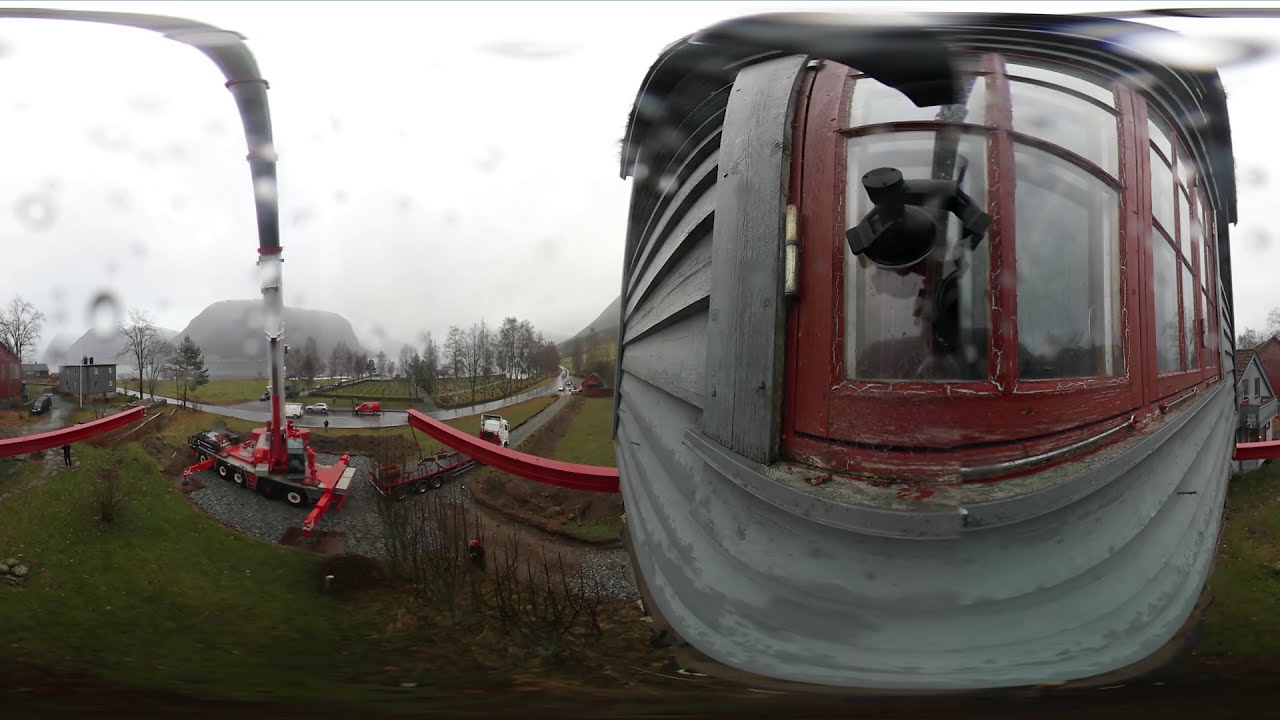The image depicts a close-up shot of a vintage, weathered construction crane, possibly part of a mecca or vehicular lifting device. The focal point is a metallic gray mechanism with horizontal lines and a curved front, situated on the right-hand side of the horizontal rectangular frame. Emerging from a red-trimmed window in the center is a black cylindrical object, complemented by a red metal bar extending from the rear. The crane stands on a flatbed trailer, supported by a substantial metal arm that stretches skyward before bending over. The scene, set in a verdant park area, showcases green trees and grassy areas interspersed with roads and distant buildings that appear gray due to the blurred background. Raindrops suggest recent rain, under a gray, overcast sky. Additionally, there are distant cars and a white tractor trailer visible on the roads, contributing to the overall sense of a rainy, quiet construction site devoid of people or animals.